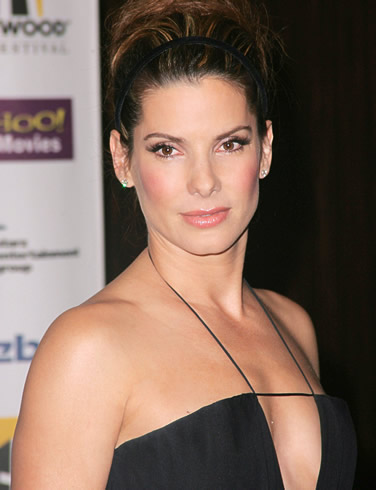In this indoor photograph, actress Sandra Bullock is featured from just below the chest upward, suggesting the setting is likely an event, possibly a movie premiere. Sandra, a Caucasian woman with brown hair pulled up into a high ponytail and secured with a black headband, displays a sophisticated appearance. She dons a black strapless dress with a deep V-cut that reveals a notable amount of cleavage. The dress has a thin strap around her neck and a thin horizontal strap that connects the bust area. Her shoulders are bare, and she accessorizes with earrings; one is a small, clear gemstone, while the other has a greenish tint. Her makeup includes heavy mascara, blush, and pink lipstick. In the background, a dark brown or black curtain occupies the right-hand side, while on the left-hand side, there is a banner featuring various logos, one of which is identifiable as Yahoo! Movies. The overall atmosphere and details suggest it is a promotional or significant event.